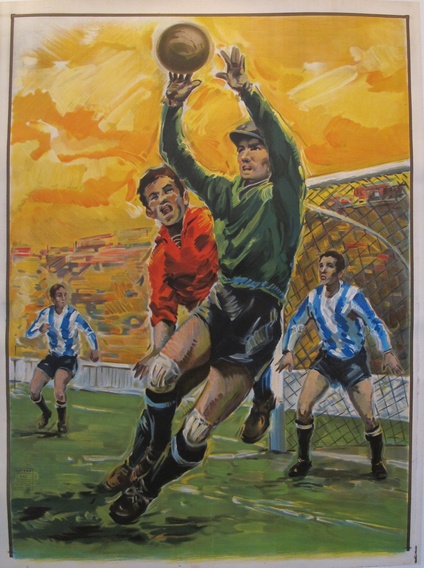The image depicts a vintage, illustrated scene of four men on a green field, engaged in a sport that combines elements of basketball and soccer. The field features a white stripe and a goal in the right background. The sky is painted yellowish, suggesting late afternoon light. The background shows a white wall and a crowd depicted in abstract yellow, red, and brown tones, making it hard to discern individual people.

The players are dressed in an eclectic mix of uniforms. Two players wear long-sleeved white tops with black vertical stripes, black shorts, and black socks, suggesting a classic soccer outfit. The player standing in the goal area appears to be the goalie. In the foreground, one player in a long-sleeved green top, black shorts, and white knee pads has his hands up, seemingly catching or blocking a ball, which appears to be copper or bronze in color. Another player in a red top is positioned behind the green-clad player, seemingly trying to intercept the ball. The uniforms differ in colors and styles, creating an air of ambiguity about the exact sport being represented.